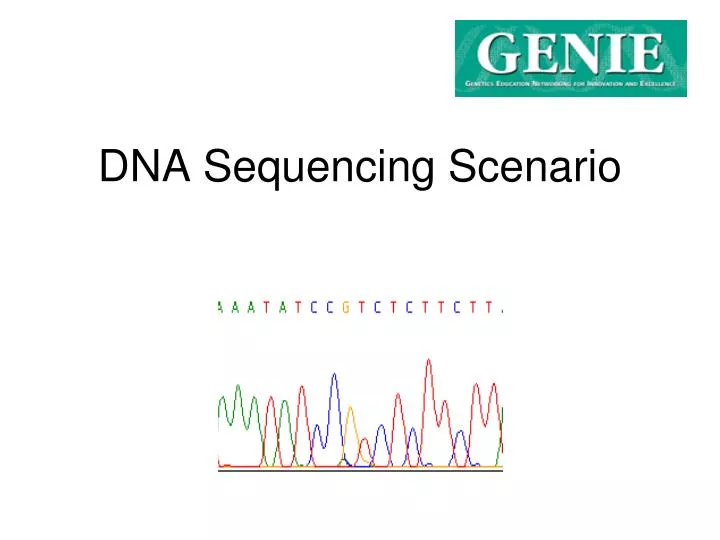The image displays a clean and detailed PowerPoint slide titled "DNA Sequencing Scenario" in black sans-serif font. Positioned in the upper right corner is a green logo with the text "GENIE" in white capital letters. Beneath the title, the slide features a graphic resembling a heartbeat monitor, with a sequence of letters—A-A-A-T-A-T-C-C-G-T-C-T—each uniquely color-coded in red, green, yellow, and blue. Corresponding to these letters, the slide includes wavy lines that mirror the colors of the letters, representing a wavelength or line graph with distinct peaks and valleys. The logo also mentions something related to genetics education, although the exact wording is blurry and indecipherable.